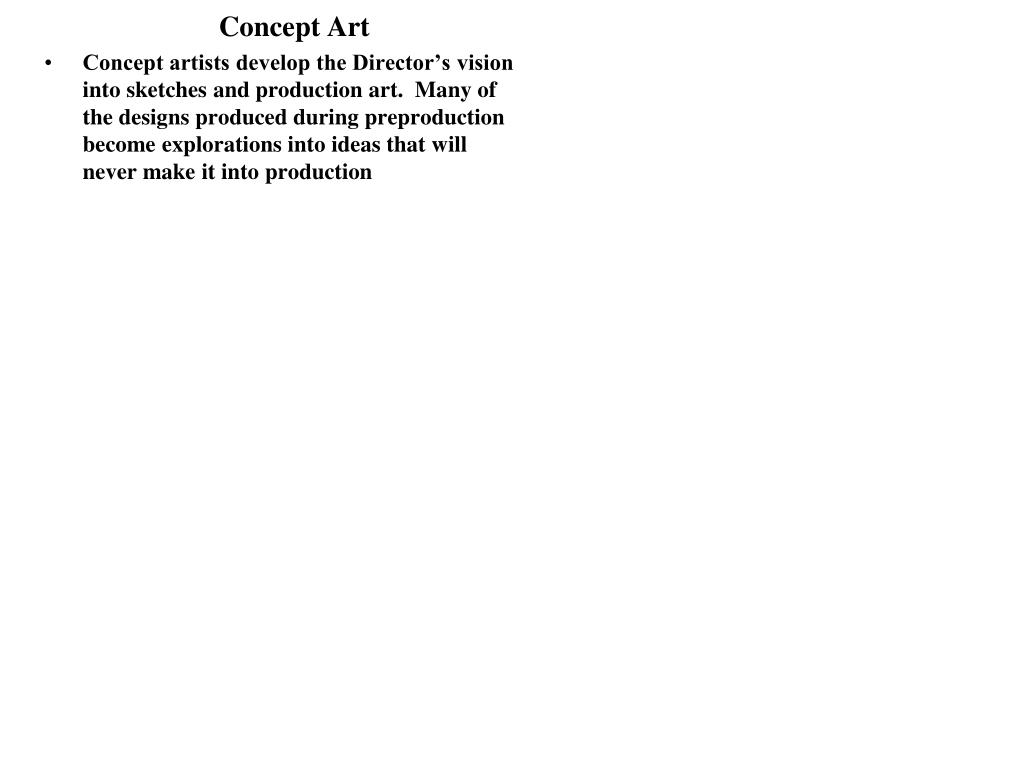The image features black, bolded text in Times New Roman on a white background. Centrally positioned at the top is a heading that reads "Concept Art," with only the initial letters capitalized. Beneath it, a single bulleted paragraph, justified to the left, states: "Concept artists develop the director's vision into sketches and production art. Many of the designs produced during pre-production become explorations into ideas that will never make it into production." Notably, there is a period after "art" but not after "production." The text is unusually condensed, occupying a small corner of the image rather than extending horizontally across the entire view.